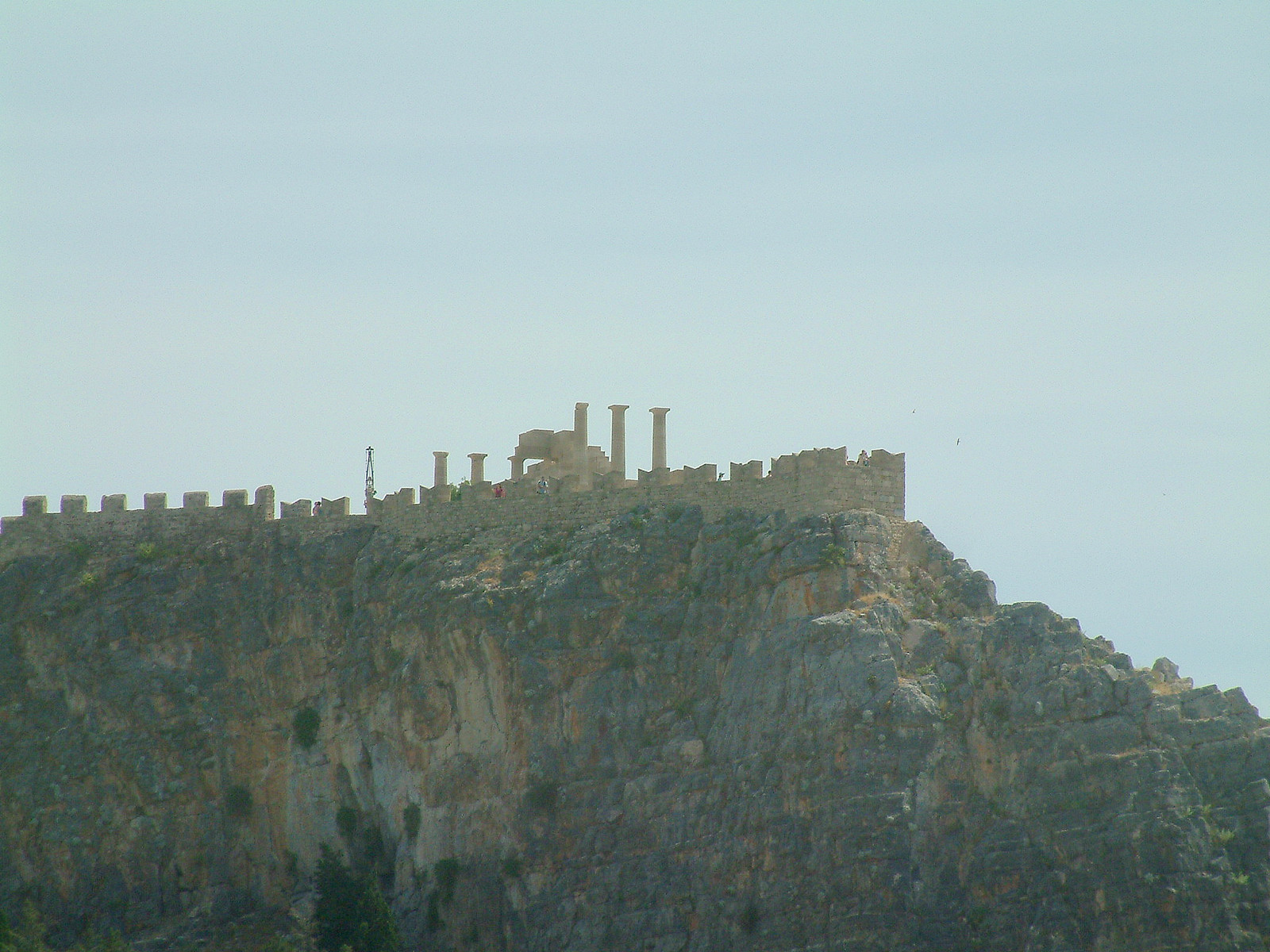The photograph captures a rugged, rocky cliff, its jagged gray and tan surfaces adorned with patches of green moss and sporadic growths of trees and shrubs. Atop the cliff stands an ancient, stone structure resembling a castle, marked by high pillars and encircled by a wall. This structure features four prominent columns and additional posts, all of which are a cohesive, weathered shade of tan or white. The backdrop is a light blue sky, punctuated with white clouds, suggesting a foggy day, though the sun can still be seen shining. The overall scene exudes an ancient, timeless quality, devoid of any human presence, and the image is not signed or copyrighted.